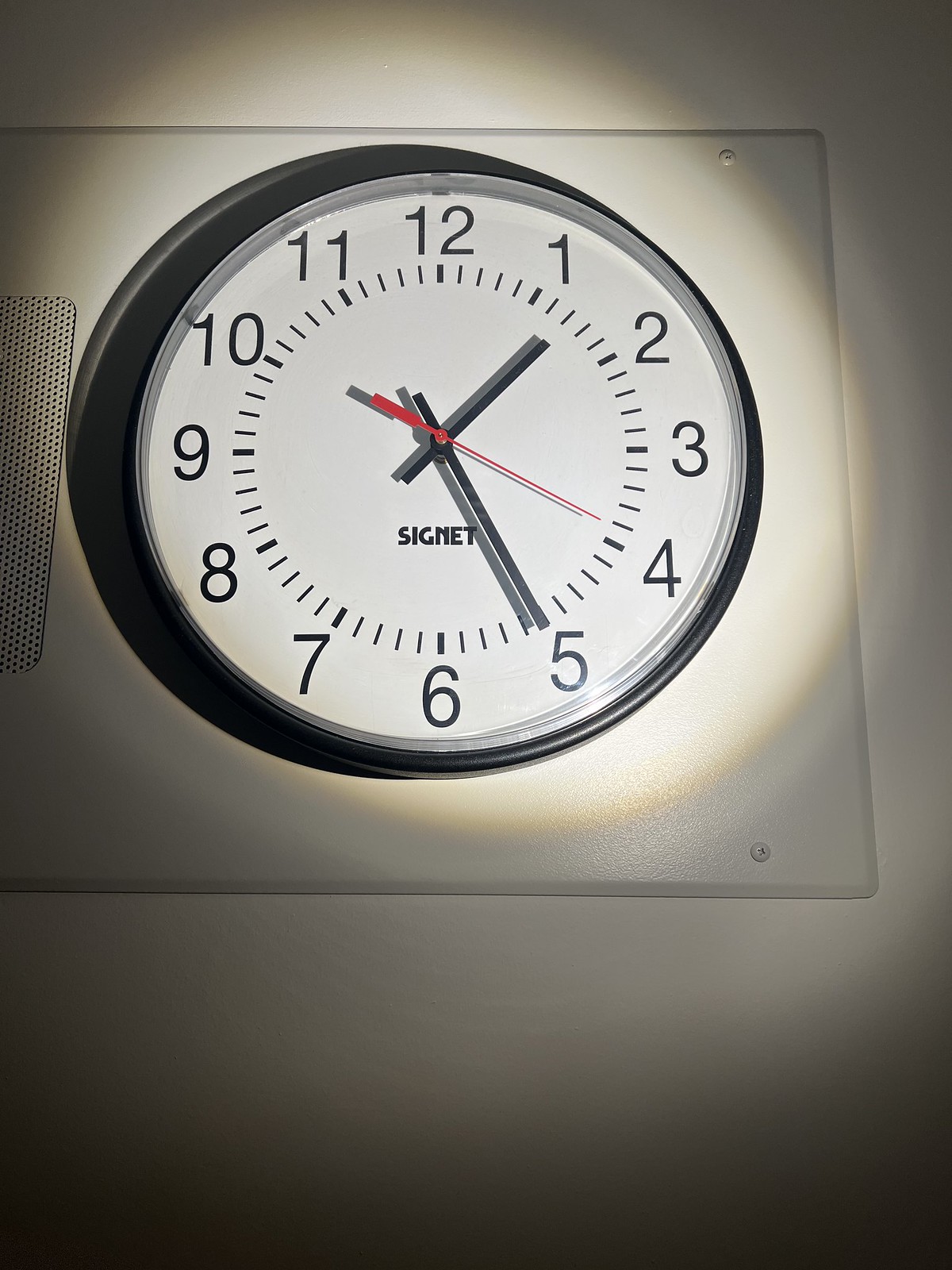This is a detailed photograph of an old-school round clock taken from a low angle, looking up. The background of the image is predominantly gray, transitioning to a darker, black hue towards the bottom corners. A strong light source shines directly onto the clock, creating a circle of illumination around it and casting a shadow on the left side. The clock is mounted on a square piece of material, possibly plastic or glass, which has small knobs near its corners, suggesting it is screwed into the tan wall behind it. The clock itself is encased in a black rim and features a white face with black numbers (1 through 12) and minute markers. The clock has three hands: a short black hour hand, a long black minute hand, and a thin red second hand. The brand name "Cignet" is inscribed below the center of the clock hands. Although there is some glare on the clock face, it mainly surrounds the clock but spares the area near the numbers 7, 8, and 9. The time displayed is approximately 1:25.